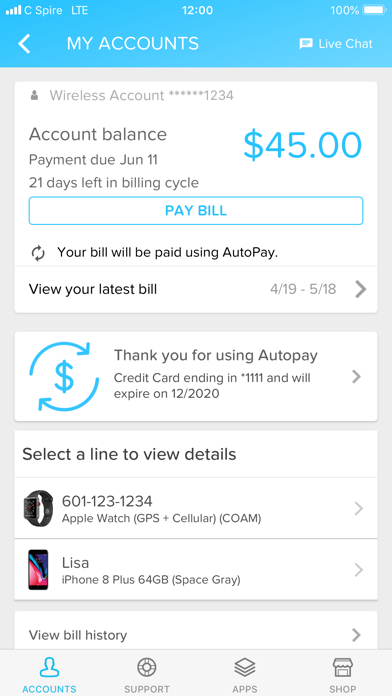The image appears to be a screenshot taken from a mobile phone. The status bar at the top indicates full signal strength with the indicators "C Spire LTE," the time "12:00," a battery fully charged at "100%," and corresponding icons.

Below the status bar, within a blue banner, there are navigation and interactive options: a left arrow, the "My Account" label, and a "Live Chat" icon.

The main content of the screenshot is centered around managing a wireless account. A rectangular box labeled "Wireless Account" displays partially redacted account details with stars substituting some numbers. It includes information such as "Account Balance" and "Payment Due: June 11th," along with a note of "21 days left in a billing cycle." To the right, the amount due is listed as "$45." Below this section, there is a prominently highlighted "Pay Bill" button in blue, followed by a refresh button and a notice indicating that the bill will be paid using AutoPay. Additionally, there is an option to "View Your Latest Bill," with the date range "4/19 - 5/18" accompanied by a right arrow.

The lower part of the screenshot includes another rectangular section with a message thanking the user for utilizing AutoPay, accompanied by an information icon involving a money symbol and a refresh arrow.

Towards the bottom of the image, there is an instruction to "Select a Line to View Details." This section lists a phone number connected to two devices: an Apple Watch and an iPhone, with the name "Lisa" associated with the iPhone.